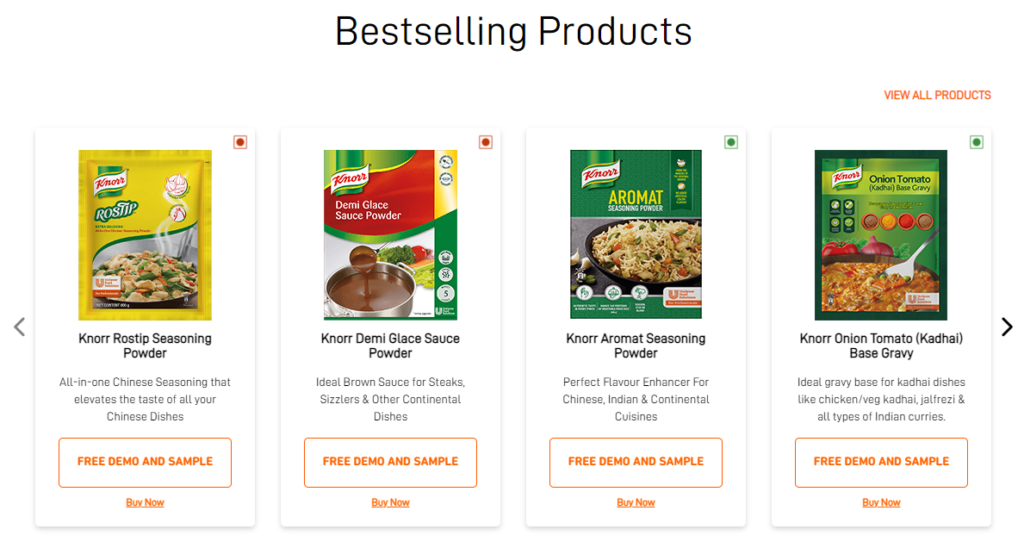The image displays a series of food items under the heading "Best-Selling Products," showcased in a grid of four rectangles. Each rectangle features a specific product with a descriptive text beneath it. Below the descriptions, there are orange-printed boxes that read "Free Demo and Sample," and at the very bottom, there's an "Buy It Now" button in orange with an underline, indicating a clickable area.

In the upper left corner, there is an option labeled "View All Products" in orange text. Each product image also includes a small, colored dot in the upper right corner of its box: the first two dots are red, and the last two are green, possibly indicating availability or status.

From left to right, the products are:
1. **Nor Roast Dip Seasoning Powder**: Described as an "all-in-one Chinese seasoning that elevates the taste of all your Chinese dishes."
2. **Nor Demi-Glaze Sauce Powder**: Marked as the "ideal brown sauce for steaks."
3. **Nor Aromat Seasoning Powder**
4. **Nor Onion Tomato Base Gravy**

Additionally, there are navigation buttons at the bottom, with the "Back" button appearing inactive and the "Forward" button appearing clickable.